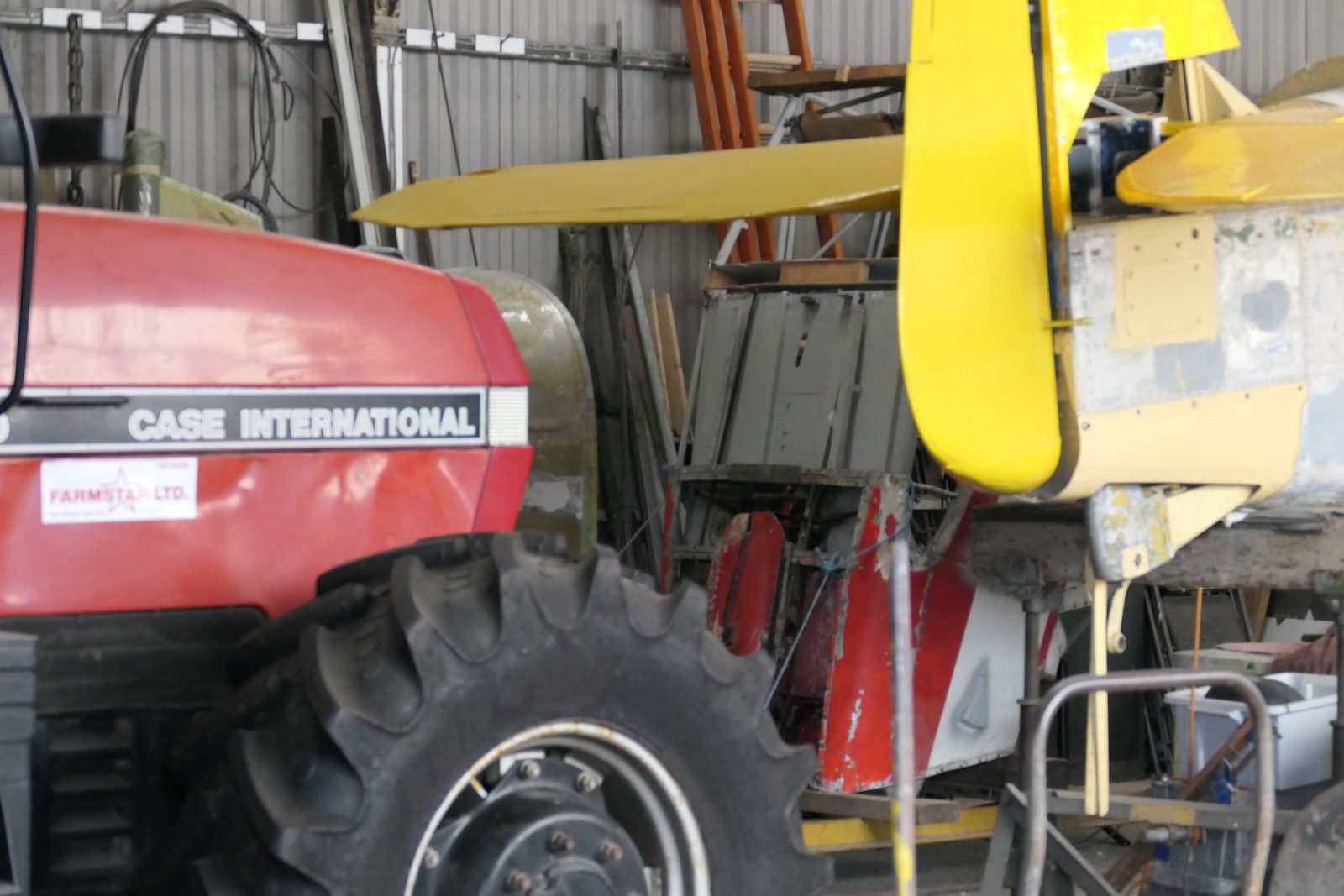This image depicts the interior of a metal shed or barn with light beige or gray walls. Dominating the left side of the frame is the front of a red Case International tractor. The tractor features large, thick wheels and displays a black bar with "Case International" emblazoned on it, along with a rectangular white sticker below that reads "Farm Star LTD." Adjacent to the tractor's front forks is a stack of various items against the wall; these include a yellow fork beneath a wooden-colored surfboard and some metal sheets. The shed also contains farming equipment, ladders, boards, and a hand truck. In the middle of the shed, there's a clutter of spare parts, including what appears to be the hood of a tractor. On the right, partially visible, is the yellow tail and ailerons of a plane, adding to the eclectic mix of items stored in the space.